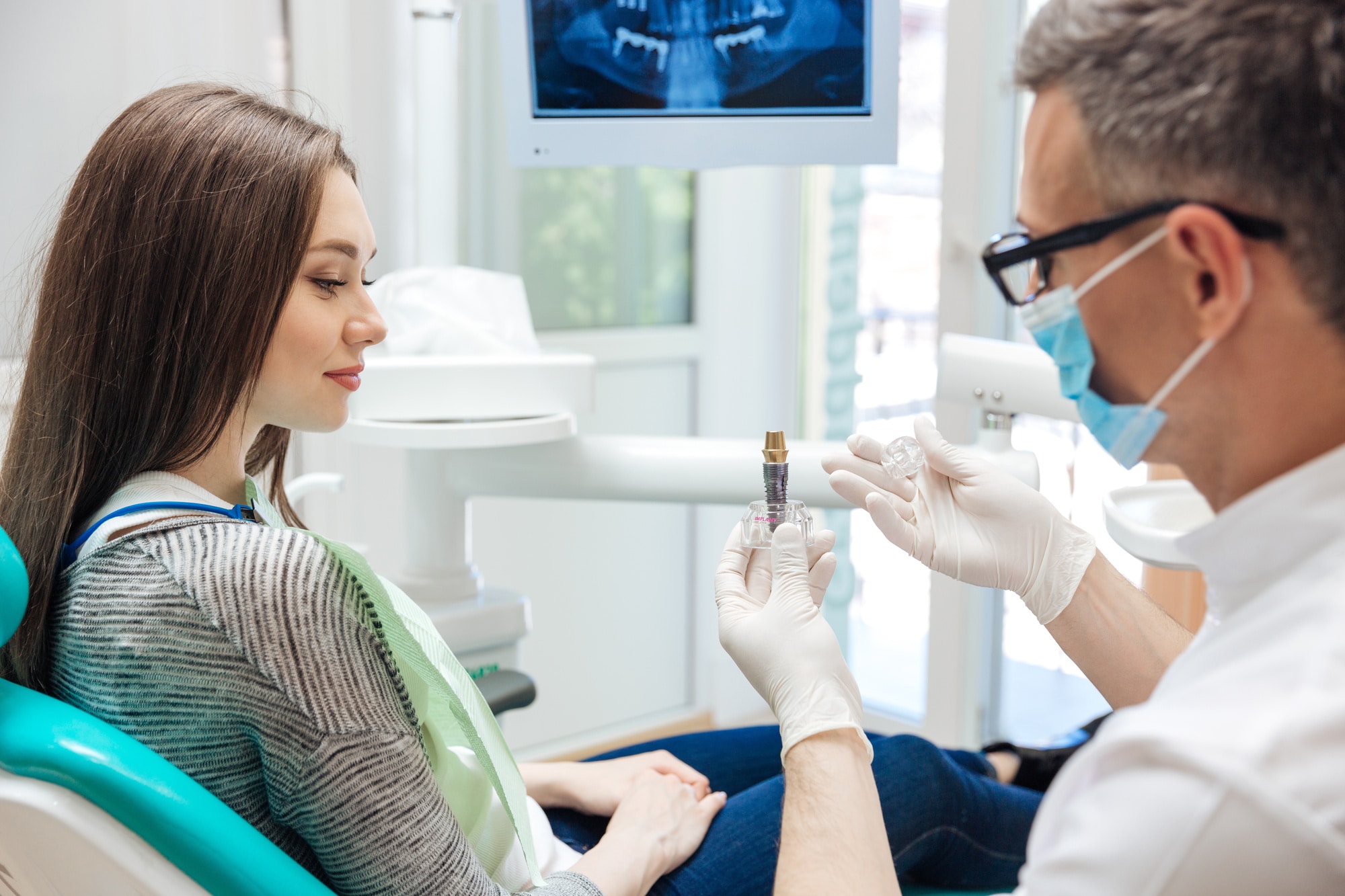The image depicts a woman in a dentist's office, seated on a dentist chair upholstered in white and topped with a headrest. She has long, dark brown hair and is dressed in blue denim jeans that resemble leggings, paired with a brown and beige striped shirt. Draped around her neck is a green disposable dental apron. The dentist, identifiable by his white shirt and high collar, is wearing black-rimmed glasses, gray hair, latex gloves, and a blue and white surgical mask. He holds a dental tool, which appears to be partly gold and silver, contained within a clear dish. In the background, there is white dental equipment, including a monitor displaying a partial X-ray image of teeth, presumably belonging to the patient. The setting is further complemented by a window that offers a scenic view for the patient.